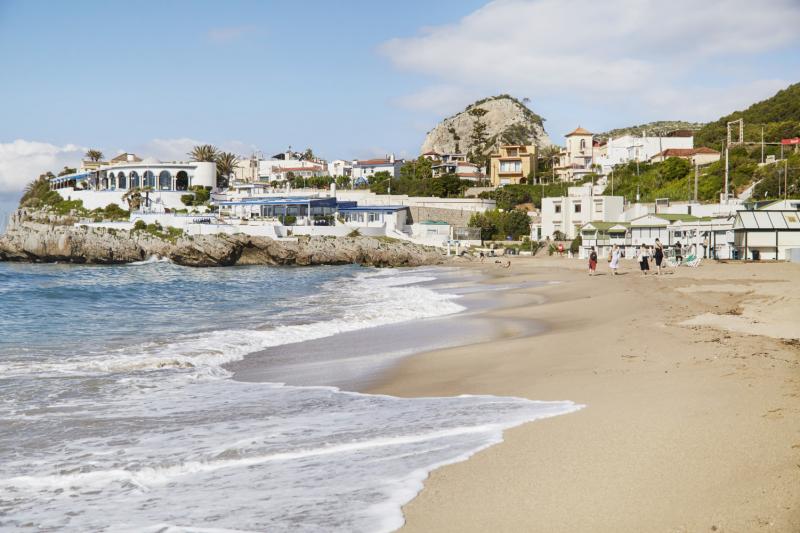The image captures a serene beach scene during a sunny day. On the right side, there is tan sand while the left side features clear, blue water with teal tints. The sea waves gently lap against the shore, contributing to the tranquil ambiance. The sky is a light blue adorned with faint, white clouds. In the background, there is a small town with predominantly white buildings, some of which appear to be beach resorts situated on a hill covered with green trees. A large, light gray stone hill stands prominently in the center. Scattered sparsely along the beach, small figures of people are visible, emphasizing the peaceful nature of the setting.